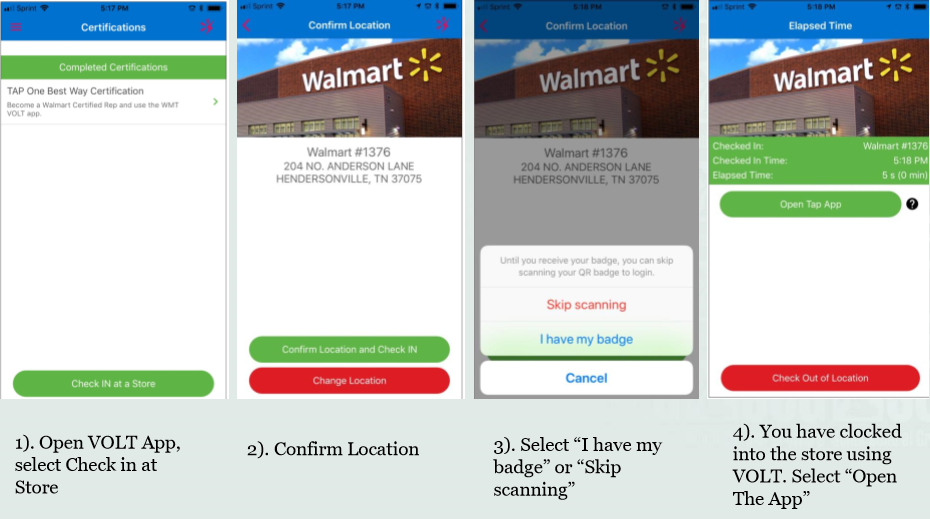This image displays four cell phone screenshots related to Walmart's check-in process.

1. The top half features a picture of a Walmart store, setting the context as a Walmart location.
2. On the right, there are three screenshots:
   - The left screenshot is labeled "Certifications." It features a green bar indicating "Completed Certifications" and below it says "Tap on Best Way Certification."
   - At the bottom of each screenshot, there are steps guiding through the check-in process:
     - Step 1: "Open Vault app, select check in at store."
     - Step 2: "Confirm location."
     - Step 3: "Select 'I have my badge' or 'Skip scanning.'"
     - Step 4: "You have clocked into the store using Vault. Select open the app."
   - Notably, all screenshots show a consistent time of 5:17 PM.